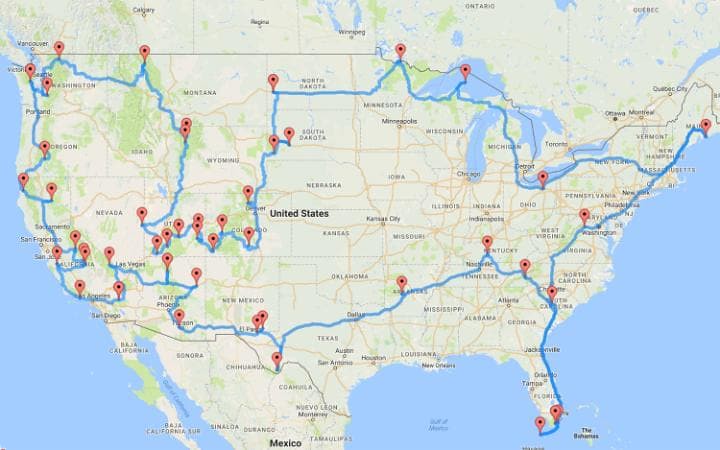This topographical map of the United States, likely sourced from a digital platform like Google Maps, visually depicts a comprehensive blue route traversing the nation. The route starts in the upper right corner of Maine, proceeds through the Midwest, reaches Seattle, Washington, and winds its way down through Nevada, California, and Texas, ultimately circling back to the tip of Florida. This blue line weaves through the outer edges and internal regions of the continental U.S., occasionally dipping into parts of Canada and Mexico. The path includes sharp angles and zigzag patterns as it navigates various states, marked by numerous red dots that designate specific waypoints. These markers punctuate major locations, including the coasts of Florida, through New York, around the Great Lakes, and into places like Las Vegas and Seattle, among others. The entire route meticulously charts a course around the outer expanse, through the central corridors, and along the coastlines of the U.S., highlighting many significant stopping points with vibrant red dots.